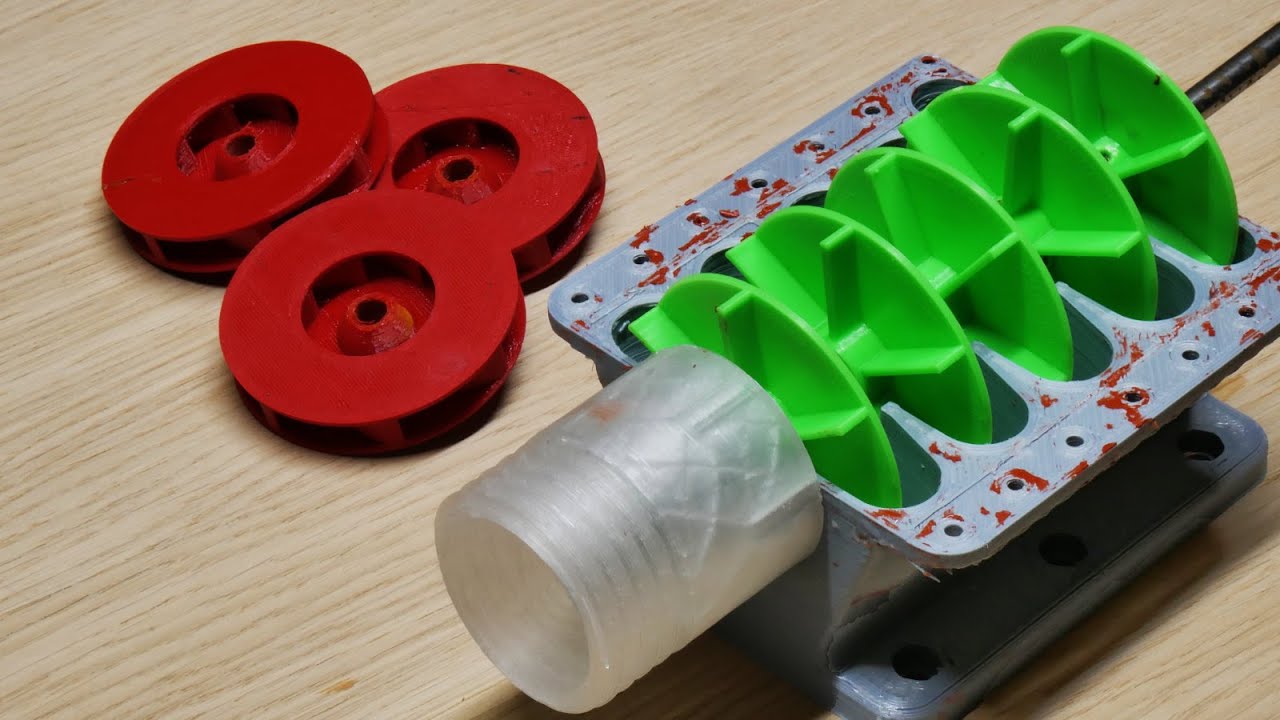The image depicts a light brown wooden table or workbench on which a mechanical setup is displayed. On the top left of the table, there are three small, dark red, fluted-edge discs with central holes, possibly designed to fit onto a shaft or similar mechanism. To the right, a gray metal contraption is visible, featuring five channels, each containing a green, wheel-like disc. These green discs are aligned in a row and appear to rotate around a central metal shaft extending from the upper right side of the contraption. Additionally, this setup includes a translucent gray-white cap positioned at the bottom left of the gray metal object. The overall setting suggests a collection of components possibly related to machinery or tool parts, although the specific function of these parts remains unclear. Red splatters and splotches can be seen on the metal piece, adding to its mechanical and utilitarian appearance.